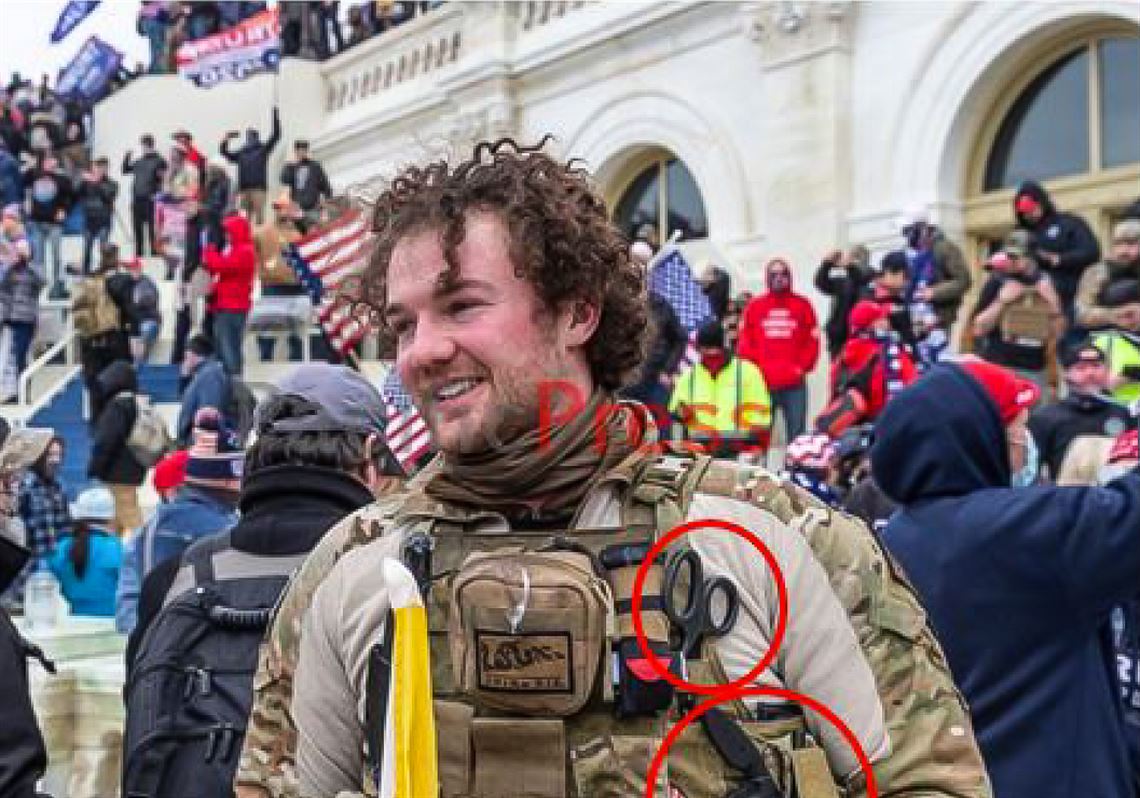The photograph, digitally enhanced and in full color, captures a scene outdoors on an overcast and chilly day, likely at a rally or protest during the January 6th events at the U.S. Capitol. The square image prominently features a man at the center, distinguished by his military fatigues. He is wearing a vest laden with pouches and gadgets, including a pair of black scissors circled in red, and a label with the word "PRESS" in red text. He has thick, curly brown hair, a beard, and stubble, indicating he isn't active duty military. The background reveals a white government-style building with distinctive arch-shaped windows and balconies with people holding signs in red, white, and blue, some of whom are also standing on the steps and ground below. The crowd, bundled in coats, sweatshirts, and caps, waves American flags and Trump banners, adding to the atmosphere of the event.